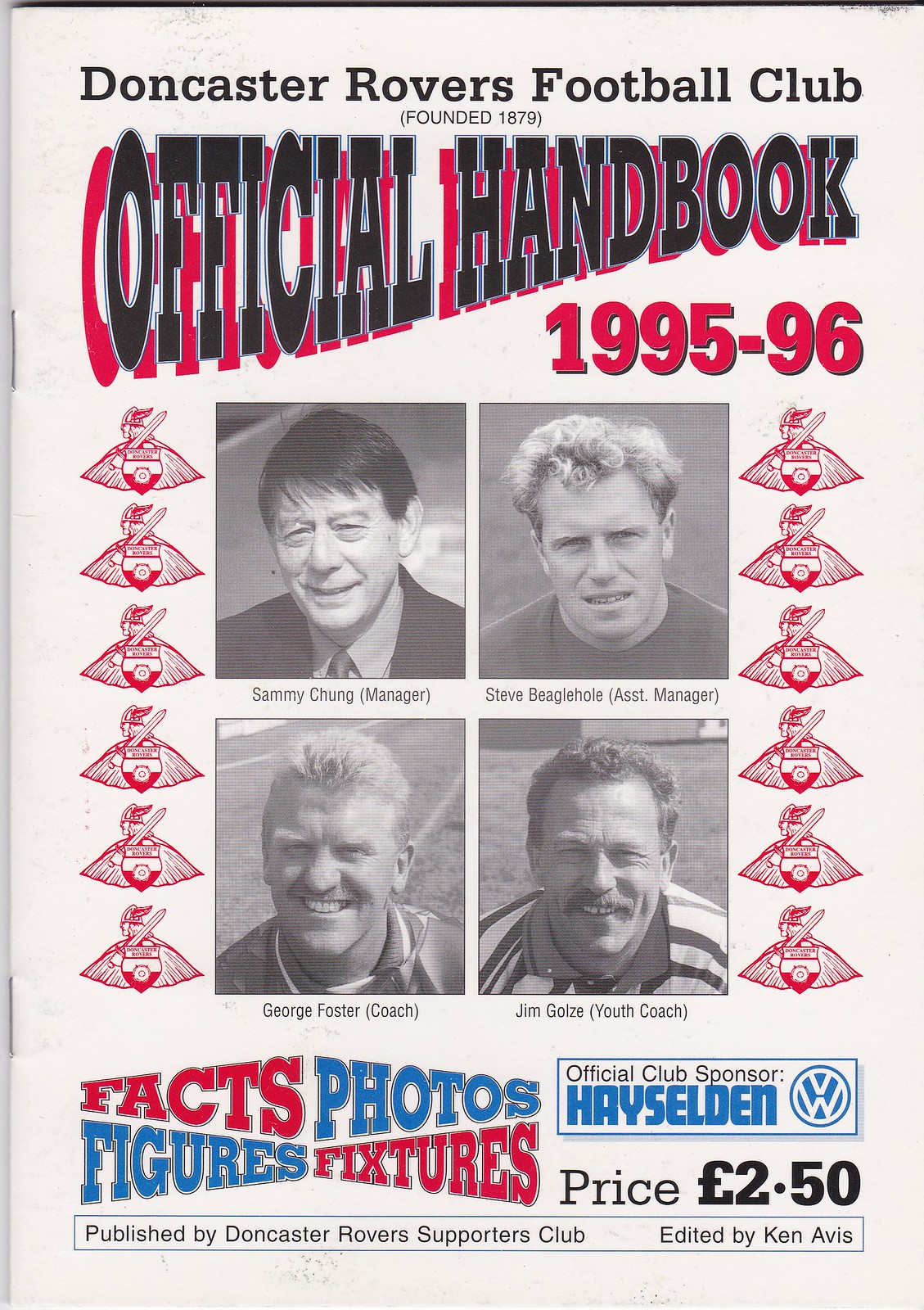The image is a photograph of the outer cover of the official handbook of Doncaster Rovers Football Club for the 1995-96 season. The background is white, and the cover is stapled on the left side, resembling a booklet. At the top, in prominent red and black lettering, it says "Official Handbook." Below this, the years "1995 to 96" are displayed in red. Centrally, there are four black-and-white portrait photographs of key personnel: Sammy Chung (Manager), Steve Beaglehole (Assistant Manager), George Foster (Coach), and Jim Golsey (Youth Coach). Along both sides of these photographs, red Doncaster Rovers logos are printed. The bottom of the cover features a rectangle with the text, "Published by Doncaster Rovers Supporters Club," edited by Ken Avice. There's also a mention of the official club sponsor, Hazelden, with the Volkswagen logo. Additionally, the price, £2.50, is indicated. The cover further highlights key contents like "Facts, Figures, Photos, Fixtures," with a mix of red and blue text.